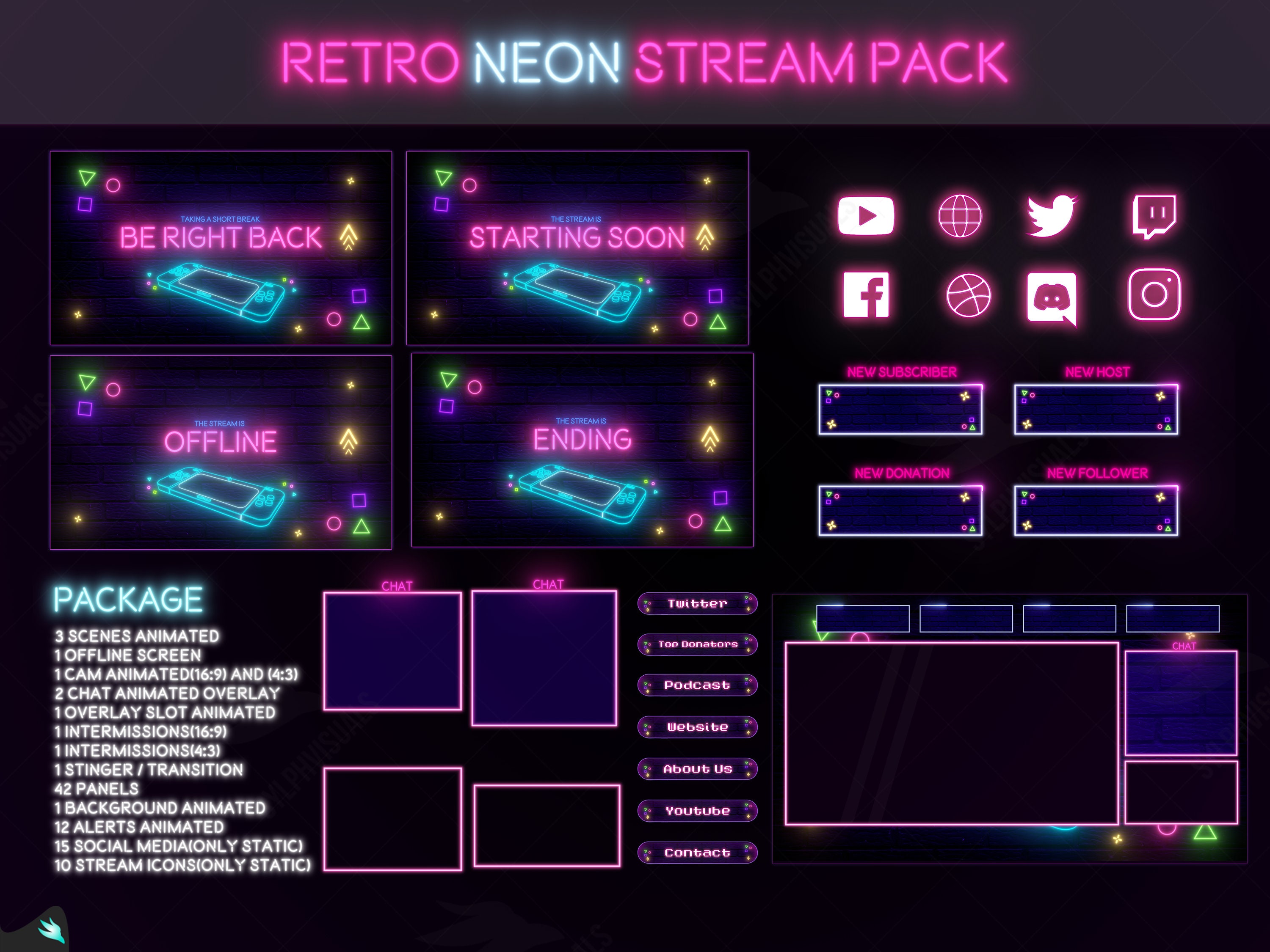The image is a highly contemporary poster titled "Retro Neon Stream Pack," showcasing a vibrant array of neon-themed visual elements against a very dark purple or black background. Neon fonts, primarily in striking pink colors, highlight various features and descriptions. On the upper left-hand side, there are four neon-outlined boxes labeled "Be Right Back," "Starting Soon," "Offline," and "Ending." Icons for popular social media platforms like Facebook, Twitter, and Instagram are prominently displayed on the right side, indicating that this streaming system is compatible with these applications. 

In the central portion of the image, there is detailed information about the different types of packages available in the stream pack. One notable package is highlighted in blue and white, detailing offerings such as two chat animated overlays and one overlay slot animated. Below this description are several blank, neon-outlined boxes, which seem designed to be chat boxes for users to interact and learn more about acquiring the pack. The dark background enhances the vibrancy of the neon colors, making the detailed descriptions and various icons vividly stand out, creating an eye-catching and informative visual experience.